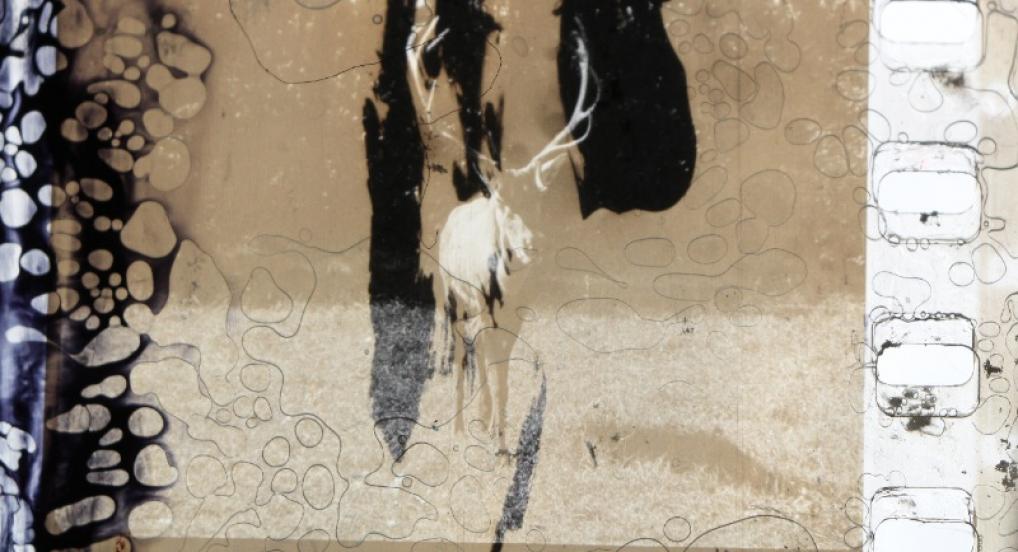The image depicts a detailed and captivating artwork that blends elements of abstract and representational styles. Centrally positioned is an elk, characterized by large antlers, predominantly white in color. The elk stands out yet intriguingly blends into the diverse background. The upper half of the artwork features a tan color, transitioning to a lighter tan in the lower half. The left-hand side of the image presents a wave of black with tan bubbles rising through it, giving a sense of movement. The right-hand side features a white and mauve bar alongside what appear to be almost square glass blocks and more bubbles. The background is a complex mix of shapes and colors, including blacks, browns, and a white strip on the right. Overall, the elk appears somewhat ethereal and almost in shadow, juxtaposed against the abstract textures and patterns, adding to the painting's intriguing and somewhat mysterious nature.